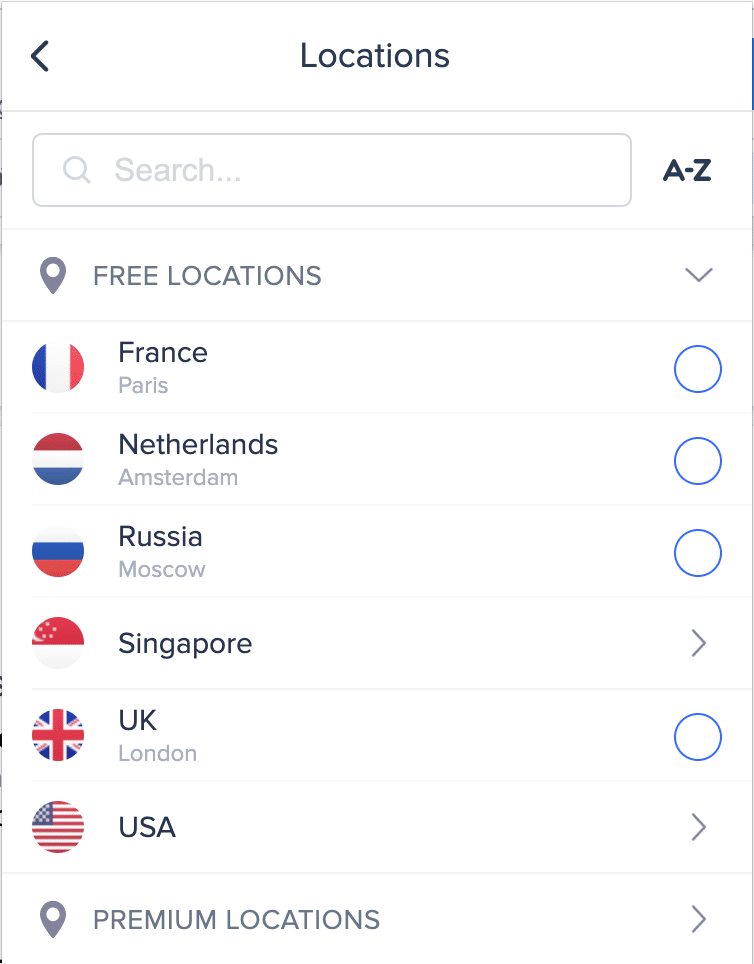The background of the screen is completely white. On the left-hand side, there is the end of a black arrow. In the center of the screen, the word "Locations" is displayed in black, followed by a thin gray line that extends horizontally across the screen.

Below this line, there's a white rectangle with a gray border containing a gray magnifying glass icon and the word "Search" in gray with an ellipsis. On the right-hand side, in bold black text, it says "A-Z," separated by dashes. Another thin gray line stretches across the screen, mirroring the one above.

In all capital letters and in gray, "THREE LOCATIONS" is written, with a downward-pointing arrow on the right side in black. Another thin gray line appears below this.

A blue, white, and red circle representing the France flag is displayed, with "FRANCE" in black beneath it and "Paris" in gray below that. Adjacent is another blue circle outlined in blue with a white interior. A thin gray line separates this section, followed by a circle representing the Netherlands flag in red, white, and blue. Below it, "NETHERLANDS" is displayed in black, with "Amsterdam" in gray beneath it. A matching blue circle is present, followed by another thin gray line.

Next, a circle depicts the Russia flag, with "RUSSIA" in black and "Moscow" in gray below it. There's a similar blue circle, then another thin gray line. A symbol resembling a signal board features a red top half and a white bottom half, with a gray arrow pointing right. 

Following this, there's a circle showing the UK flag with "UK" and "London" in black beside it, and a similar blue circle again. Lastly, "USA" is accompanied by the USA flag and a gray arrow pointing to the right. At the bottom, the text "PREMIUM LOCATION" is displayed.